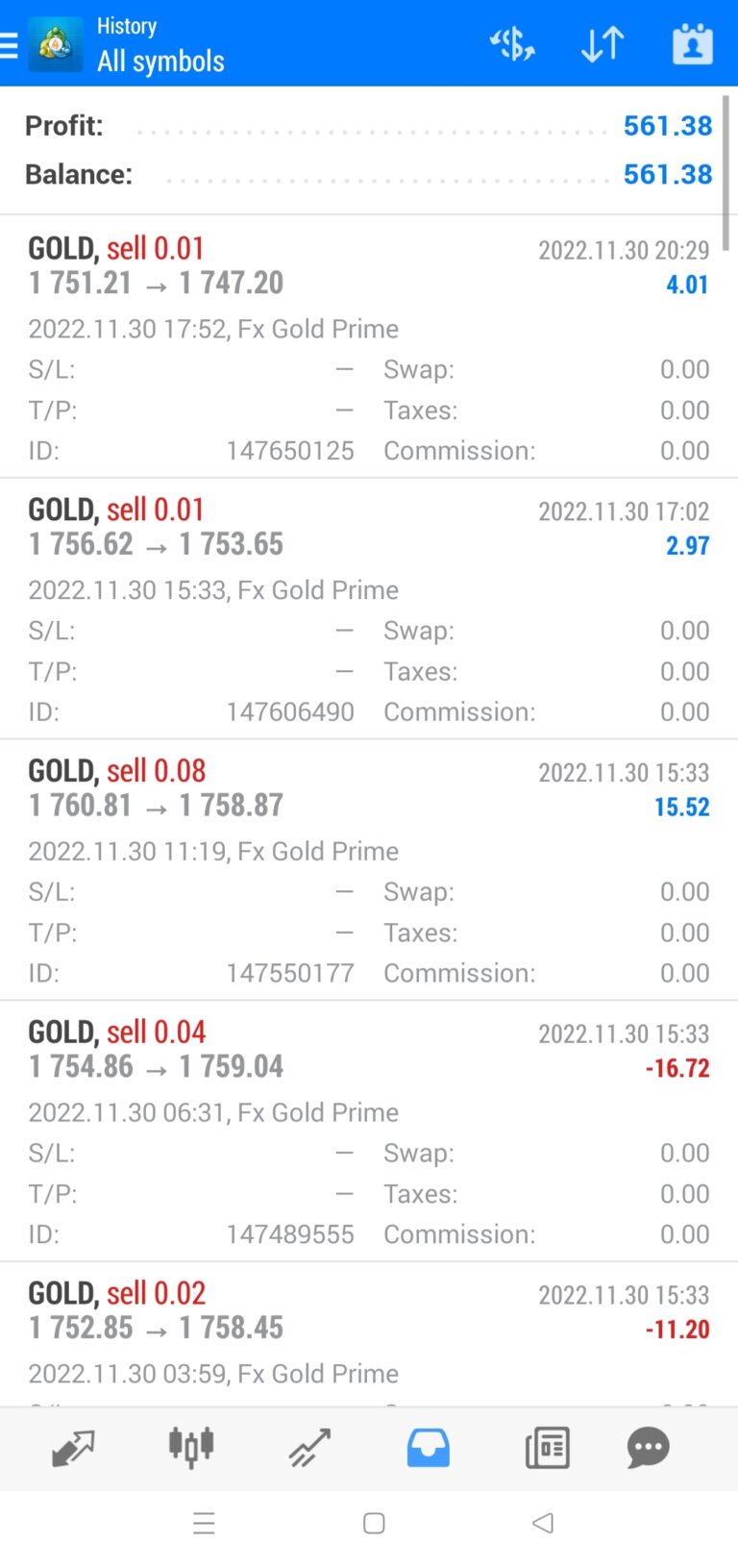This image is a detailed screenshot of an individual's trading history from a mobile trading platform, presented in a long, rectangular portrait orientation typical of a cell phone screen. The top of the screenshot features a blue horizontal navigation bar with white text, icons, and a hamburger menu to the left. Adjacent to the hamburger menu is a flower icon set against a blue background, followed by the text "History" and "All Symbols." Further to the right, a dollar sign symbol encircled by arrows in a counterclockwise rotation is visible, accompanied by calendar icons.

The primary part of the screen showcases a white background divided into informative segments. The first section summarizes the user's financial status, displaying "Profit" on the left and "56138" as both the profit and balance values on the right.

Below this summary, a list of trading activities is itemized. The entries feature various trading actions involving gold (denoted as "gold") with corresponding trade sizes (e.g., "Sell 0.01" in red text indicating transaction values). The list is organized by individual trade actions and their respective sizes and profits. Red text indicates sell transactions, and likely, profitability can be inferred based on the text color and accompanying entries.

This descriptive screenshot illustrates the user's trading activities, offering a clear and concise representation of their trading history, including profit and loss data, thus providing valuable insight into their trading performance on the platform.